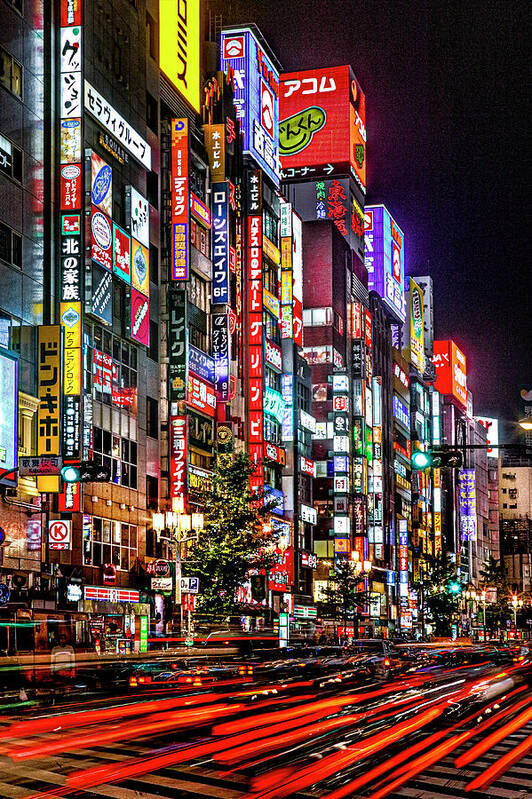This highly detailed and photorealistic oil painting captures a vibrant nighttime cityscape that appears to be set in Asia, likely in a bustling metropolis like Shanghai or Tokyo. Dominating the scene are towering skyscrapers adorned with a multitude of neon lights and advertisements, all featuring Asian characters, creating an atmosphere reminiscent of a neon-drenched Broadway. These advertisements, displayed on LCD screens and billboards, cast a colorful glow that melds various hues like red, purple, and yellow into the night sky. At the bottom of the painting, a striking time-lapse effect reveals streaks of red light from the taillights of cars zipping across the road, heading away from the viewer. The cars blur into the distance, emphasizing the speed and movement of city life. Street lights and patches of greenery, including some urban trees, are interspersed between the road and skyscrapers, providing a touch of natural contrast to the urban scene. The night sky, visible in the top right corner, forms a black canvas that enhances the illuminated cityscape below.